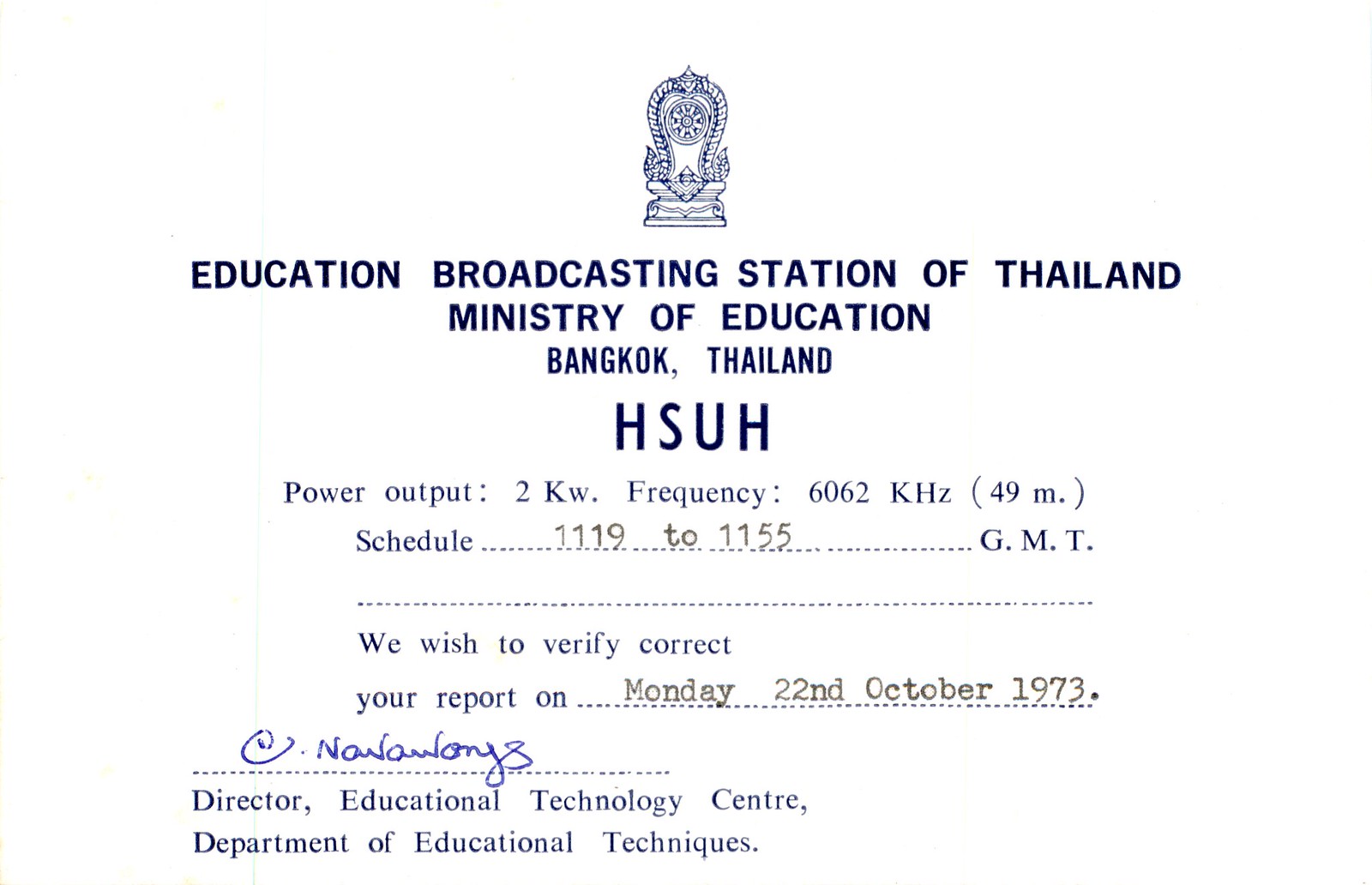The image is of a vintage QSL confirmation card, likely typed on a typewriter, used by receivers to confirm broadcast reception from the Education Broadcasting Station of Thailand, Ministry of Education, Bangkok, Thailand. The card features a white background with a faded black border, a blue symbol centered at the top, and in black, all-caps letters: “EDUCATION BROADCASTING STATION OF THAILAND, MINISTRY OF EDUCATION, BANGKOK, THAILAND.” Below this, it displays the call letters "HSUH." 

In the top left corner, typewritten information specifies the power output as "2 kilowatts" and the frequency as "6062 kilohertz (49 meters)." A section titled "Schedule" lists the broadcasting time as "1119 to 1155 G.M.T.," also typed in. Further down, it states, "We wish to verify, correct your report on" followed by "Monday, 22nd, October 1973," again typewritten. The card concludes with a signature line, under which is printed "Director, Educational Technology Center, Department of Educational Techniques."